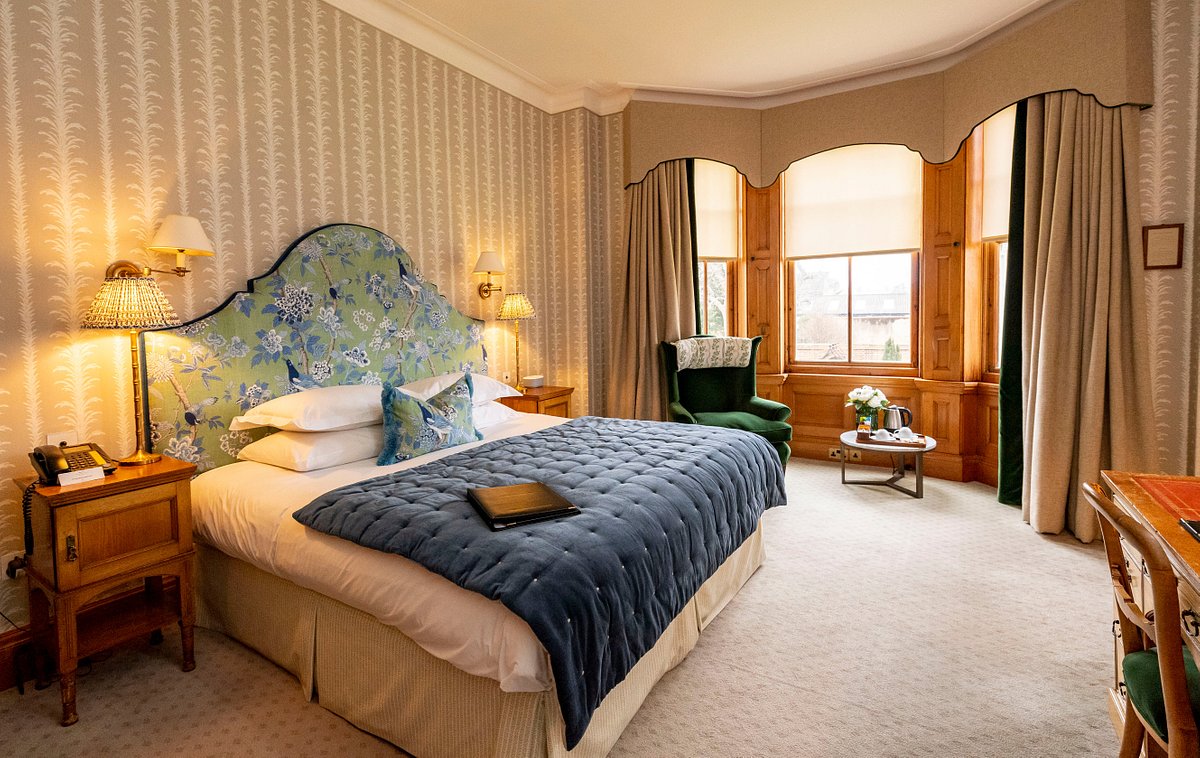This image captures an elegantly designed bedroom, which could either be a luxurious hotel room or a sophisticated personal bedroom. The color palette primarily features cream and beige tones, giving it a serene and refined atmosphere. The walls have intricate patterns, and there are rich, brown drapes adorning the large windows, which are sectioned into three panes and framed with detailed woodwork. Before the windows, there is a comfortable green armchair accompanied by a low table holding a teapot, white cups, and some flowers. To the right side of the room sits a wooden desk paired with a chair that has a green cushion. 

On the left side of the room, there is a king-size bed dressed in white sheets and adorned with four white pillows and an additional throw pillow that matches the fabric of the floral baseboard. A neatly folded blue blanket rests at the foot of the bed. Above the bed are two lamps affixed to the wall, providing soft, ambient lighting. Flanking the bed are two wooden nightstands, each with a single drawer. The nightstand on the left has a tall lamp and a telephone, while the nightstand on the right also features a lamp and a couple of decorative figures. The room's elegant décor is completed with a tan-colored rug that runs across the floor, enhancing the overall warmth and coziness of the space. The photograph was taken during the daytime, as evidenced by the ambient light streaming through the windows, although what lies beyond the windows remains a mystery.